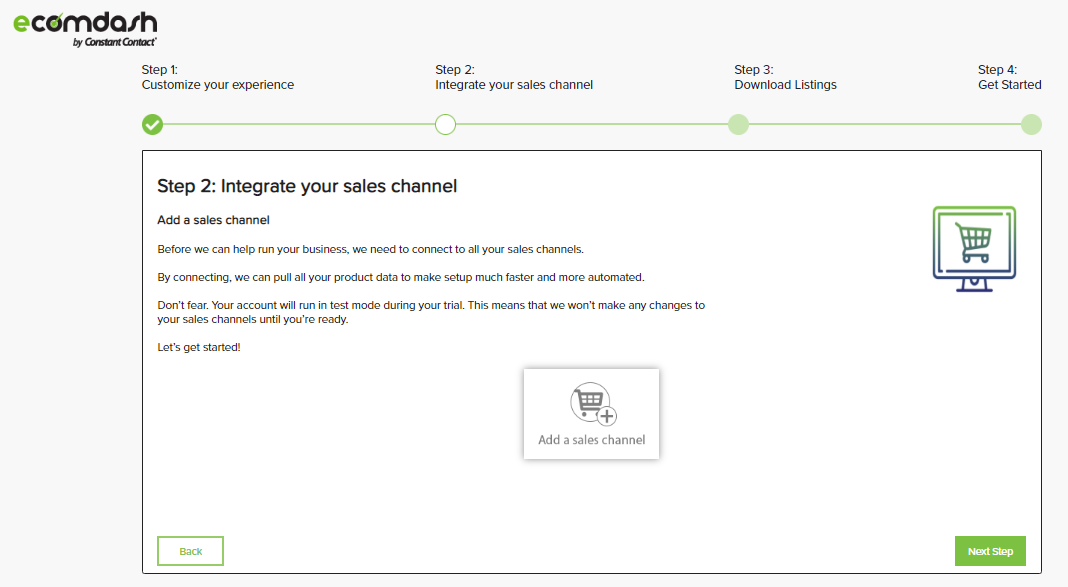Here is the cleaned-up and descriptive caption:

---

**Illustration of Ecomdash Integration Process**

The image showcases the Ecomdash interface, a tool designed to streamline business operations. Across the top of the screen, there is a four-step timeline: 1) Customize Your Experience, 2) Integrate Your Sales Channel, 3) Download Listings, and 4) Get Started. Below this timeline, a large white window pane prominently displays the heading "Integrate Your Sales Channel." 

The instructions within this pane inform the user that to efficiently run their business, they need to add a sales channel. It emphasizes that by connecting sales channels, the platform can retrieve all products and data, thereby expediting the setup process through automation. In the center of the screen, an icon featuring a plus sign invites users to add a sales channel. Additionally, a green "Next Step" button is located in the lower right-hand corner, guiding users to proceed to the subsequent step.

This interface is indicative of a versatile business operation tool aimed at enhancing efficiency through comprehensive data integration.

---